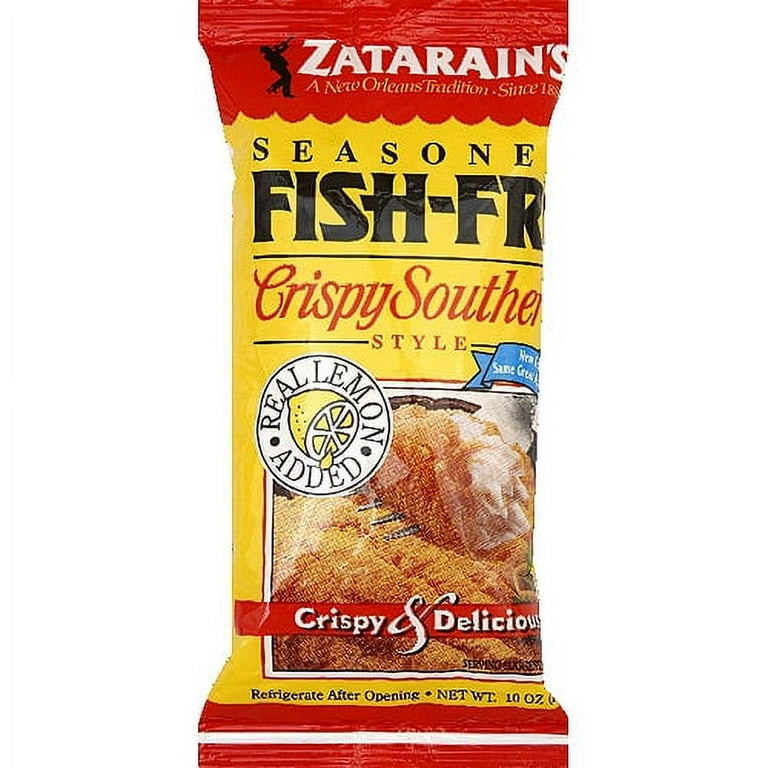The image displays a close-up of a Zatarain's Seasoned Fish Fry packaging against a completely white backdrop, accentuating the product details. The top of the bag is red with white text reading "Zatarain's New Orleans Tradition" alongside a black illustration of a trumpet player. Below this, the predominant color of the packaging is yellow, with bold black text stating "Seasoned Fish Fry." Underneath, in red text, it proclaims "Crispy Southern Style." Highlighting the flavor is a white circular badge featuring an illustration of a lemon with accompanying text that reads "Real Lemon Added." Dominating the bottom half of the bag is a low-resolution photograph displaying a fork piercing a piece of crispy, battered fish with sauce being drizzled over it. Superimposed on this image is a red bar with white text and a black shadow effect reading "Crispy and Delicious." The bottom of the bag has red arches, and small black text instructs to "Refrigerate After Opening" and notes the net weight as 10 ounces. The bag appears uneven around the edges, suggesting it was cut from a different image.